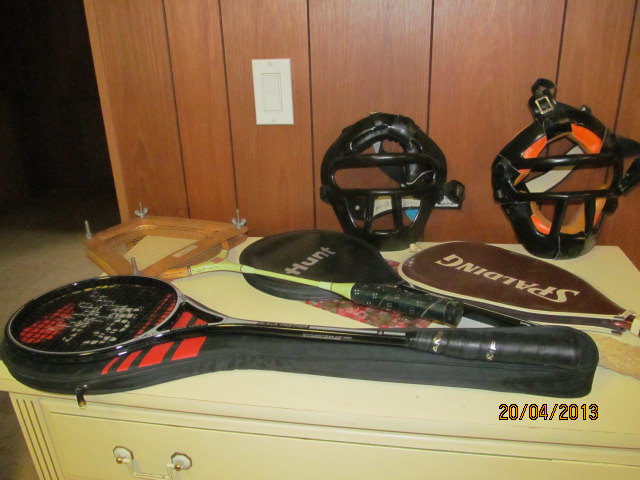The image features a medium-toned, vertically striped wood-paneled wall with a white push-button light switch. In front of the wall stands a yellowing, possibly once white, wooden dresser with a white handle on the top drawer. On top of this dresser lies a collection of sporting equipment, predominantly tennis rackets and protective masks. 

One prominent tennis racket, with a black handle and gray netting, rests on a black case adorned with red stripes. Another vintage wooden tennis racket, with a yellow handle, is encased in a classic wooden frame fastened with screws and bolts, giving it a tightened, old-school appearance. There is also a black cover labeled "Hunt," which likely contains another racket, and a brown oblong case with the word "Spaulding" in beige letters, revealing a bit of a dark pink handle.

Additionally, the image includes two face masks which appear to be catcher's or pitcher’s masks. One mask is primarily black with some orange padding, and the other is also black with similar orange accents. There's a date stamp in the bottom right corner that reads "20/04/2013," adding a dated feel to the photograph.